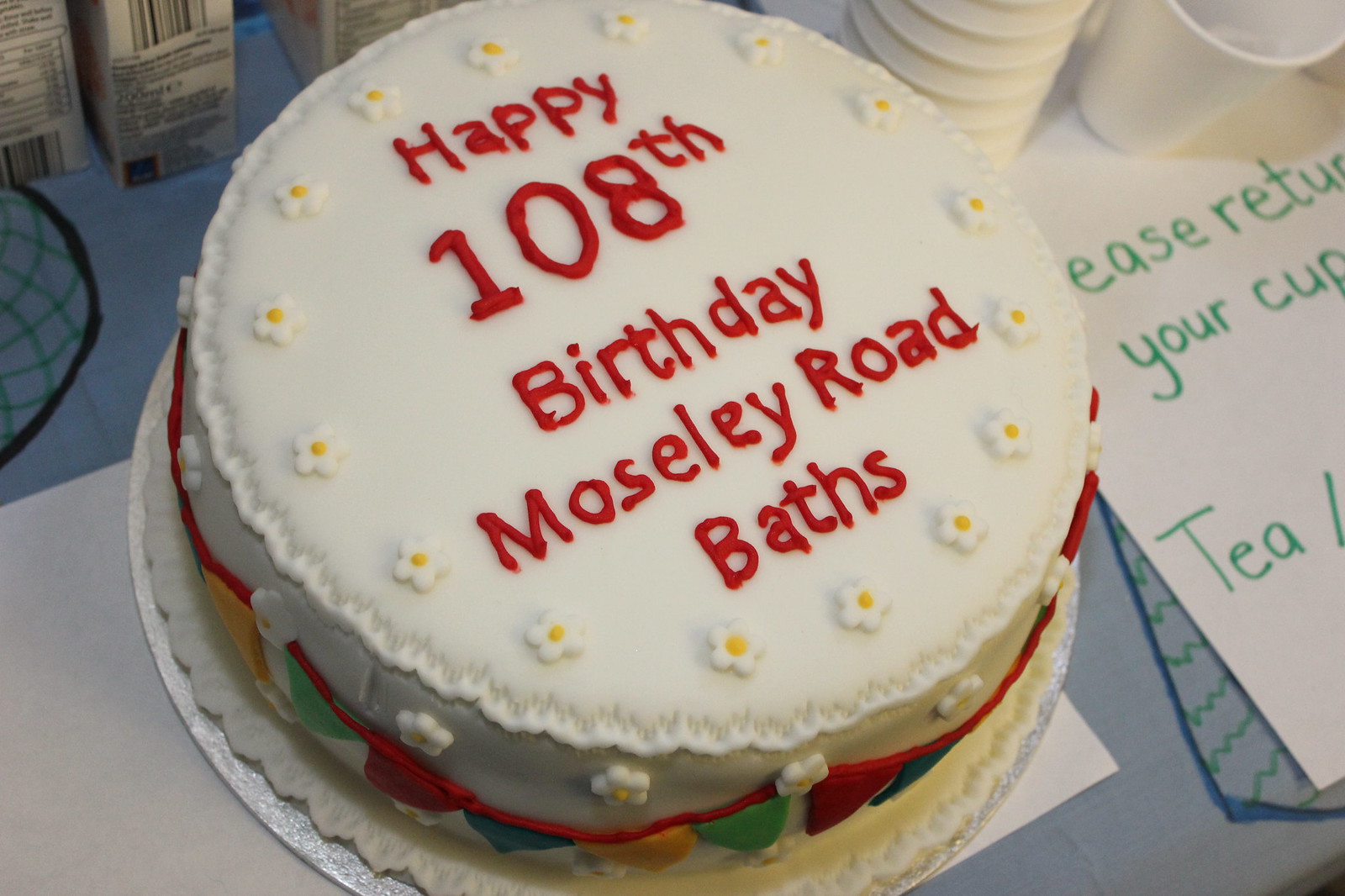The image features a round birthday cake with white icing, adorned with little daisy flowers that have yellow centers, both on top and around the sides. The cake is decorated with a festive banner of red, green, blue, and yellow flags and has a red line encircling it. Written in red icing on the top of the cake is the message: "Happy 108th Birthday, Moseley Road Baths." The cake is displayed on a round silver platter, which sits on a white table. To the right of the cake, there are stacked styrofoam cups and a green-lettered sign that reads, "Please return your cup, T slash." In the background, cartons with barcodes can be seen. The cake dominates the image, occupying most of the visual space.